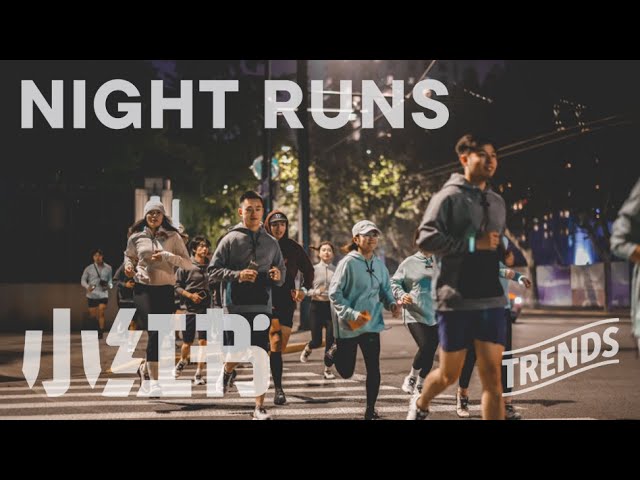This color photograph features at least thirteen young Asian men and women, likely in their late teens to early twenties, running across a dashed white-lined crosswalk at night. They are dressed in typical running attire, including shorts, hoodies, and some wearing baseball caps. The sky above them is visible, indicating it is nighttime. The background shows trees in the middle and buildings with some lit windows on the right. The rectangular image has black bars across the top and bottom, resembling a still frame from a video. At the top left, large semi-transparent white text reads "Night Runs," while the bottom left corner contains white Chinese characters. In the bottom right corner, wavy semi-transparent white text reads "Trends" with a white line above and below it.